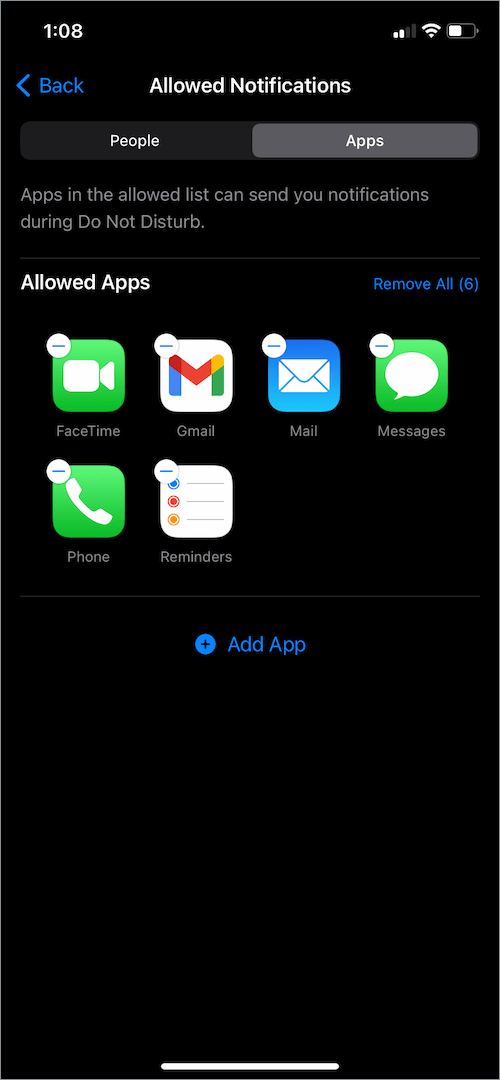A smartphone screen shows the "Do Not Disturb" settings page. At the top, a blue arrow points to the left with the number '108' displayed prominently. Below, under the "Allowed Notifications" section, the word "People" is grayed out, while "Apps" is highlighted in white, indicating that only apps are currently allowed to send notifications during Do Not Disturb mode. The phrase "Do Not Disturb" is written with initial capitalization for each word.

The "Allowed Apps" section lists six apps, as indicated by “(6)” next to the title. Each app listed—FaceTime, Gmail, Mail, Messages, Phone, and Reminders—has a minus symbol in the top-left corner, signifying that tapping this symbol will remove the app from the allowed list. A blue circle containing a black plus sign and the label "Add App" is positioned beneath the list, allowing users to add more apps to the allowed notifications list. The background of the phone interface is black, providing a stark contrast to the app icons and settings text.